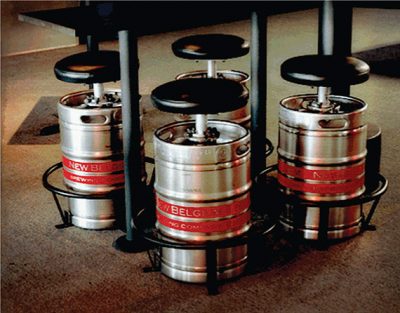The photograph depicts four metallic, silvery kegs, each outfitted with black taps or pumps on top. These kegs are strikingly shiny, hinting at their potential utility in a brewery setting, possibly connected to the New Belgium Brewery, given some barely discernible text suggesting "Belgium." Each keg has two red bands encircling its middle and handles which indicate they are designed for easy transport. They are arranged in a square formation on a gray-colored floor, possibly in a holding area with metal circular rings and poles around them. The kegs seem to be sitting slightly elevated, raising curiosity about their scale—whether they are practical beer kegs or perhaps miniaturized versions designed as barstools. The background is minimal, focused entirely on these intriguing devices, giving no other context or surrounding activities.